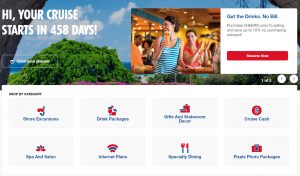An advertisement from a cruise website displays a vibrant scene at a beachside bar, featuring green trees and an idyllic shoreline in the background. A woman in a blue tank top is captured enjoying an orange drink, while another woman in a red tank top claps enthusiastically next to her. In the background, a couple looks on with interest. The website prominently announces, "Hi, your cruise starts in 458 days!," and invites travelers to explore various menu selections. The cruise packages offered include a range of options, such as different drink selections, dining choices, internet packages, cash transactions, and photo packages, all tailored to enhance the cruising experience.